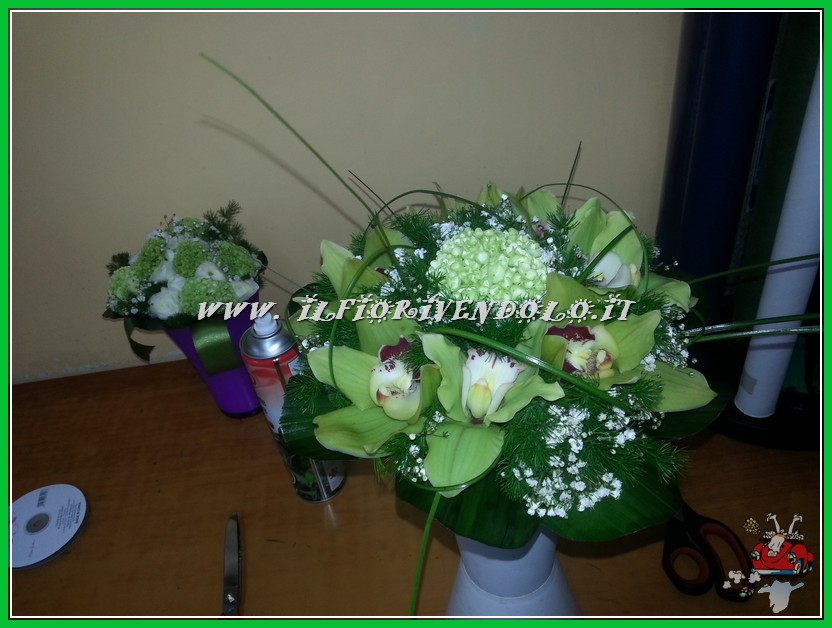The image captures an advertising photograph for an Italian florist, evident by the web address www.ilfioravendolo.it across the center of the photo. The focal point is a white jar filled with a vibrant bouquet dominated by lush green foliage. Amongst the greenery are striking purple blooms and delicate white flowers dotted throughout. Surrounding the main bouquet are various elements contributing to the scene: a spray can towards the top left, likely for flower maintenance, and another vase with similar arrangements in the background. The bouquet rests on a sturdy brown wooden table, where additional items like a white CD, a roll of ribbon, and two pairs of scissors—one partially visible, the other with its handle peeking out—reside. At the bottom right corner of the image, a whimsical red Volkswagen Beetle drawing with comical feet protruding upwards adds a playful touch. The photograph, illuminated with flash, highlights the central bouquet while subtly toning down the surroundings.